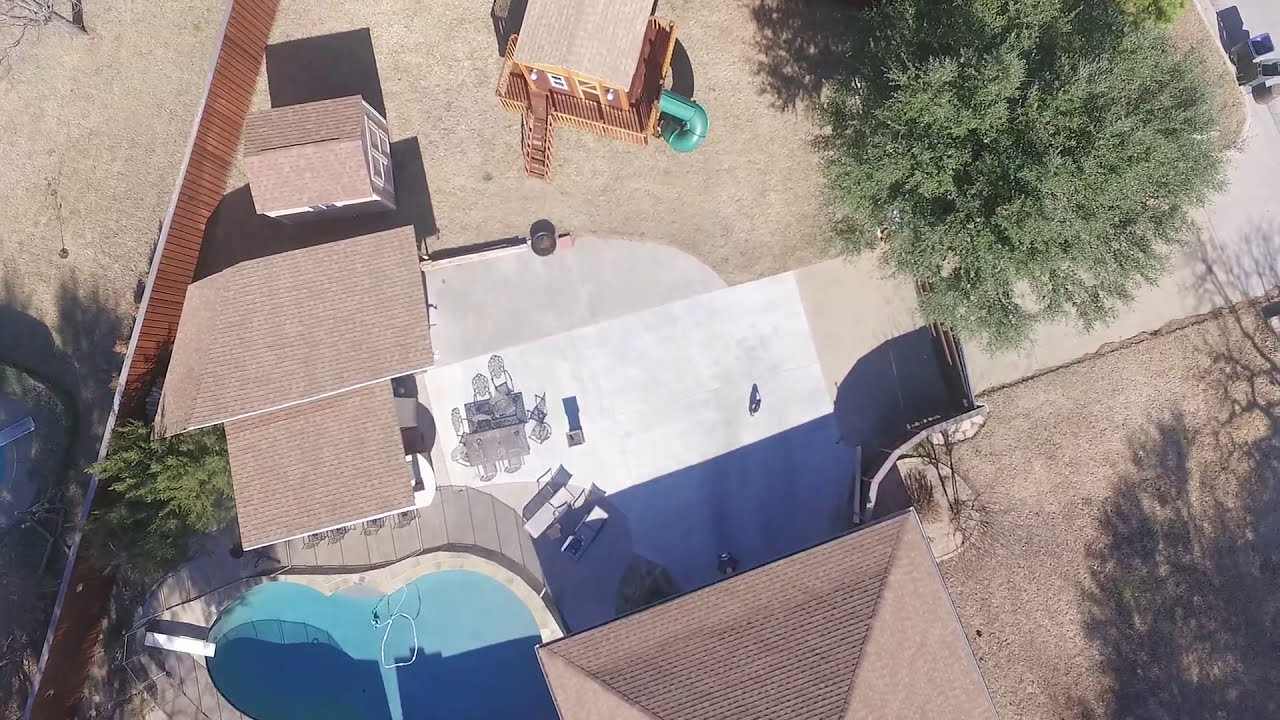This full-color aerial photograph, taken outdoors on a sunny day from an altitude of approximately 50-60 feet, captures an intimate view of someone's home and yard. Dominating the scene is a house with brown shingles, positioned centrally at the bottom of the image. The foreground features a well-manicured yard, punctuated by various objects and activity spaces. In the upper right corner, the shadow of a large green tree adds a natural touch. The center of the photograph highlights a child's play area—a barn-like structure with an adjoining deck, stairs, and a distinctive blue curved slide. Off to the left, there is a sturdy shed, colored gray, standing behind a small swimming pool. Adjacent to the pool, a table with chairs and a couple of lawn chairs are arranged, suggesting a space for relaxation and sunbathing. The palette of the image includes vivid greens, blues, browns, grays, off-whites, and blacks, indicating a vibrant, well-used outdoor space. Overall, the photograph presents a detailed and structured backyard environment, bathed in the light of midday.